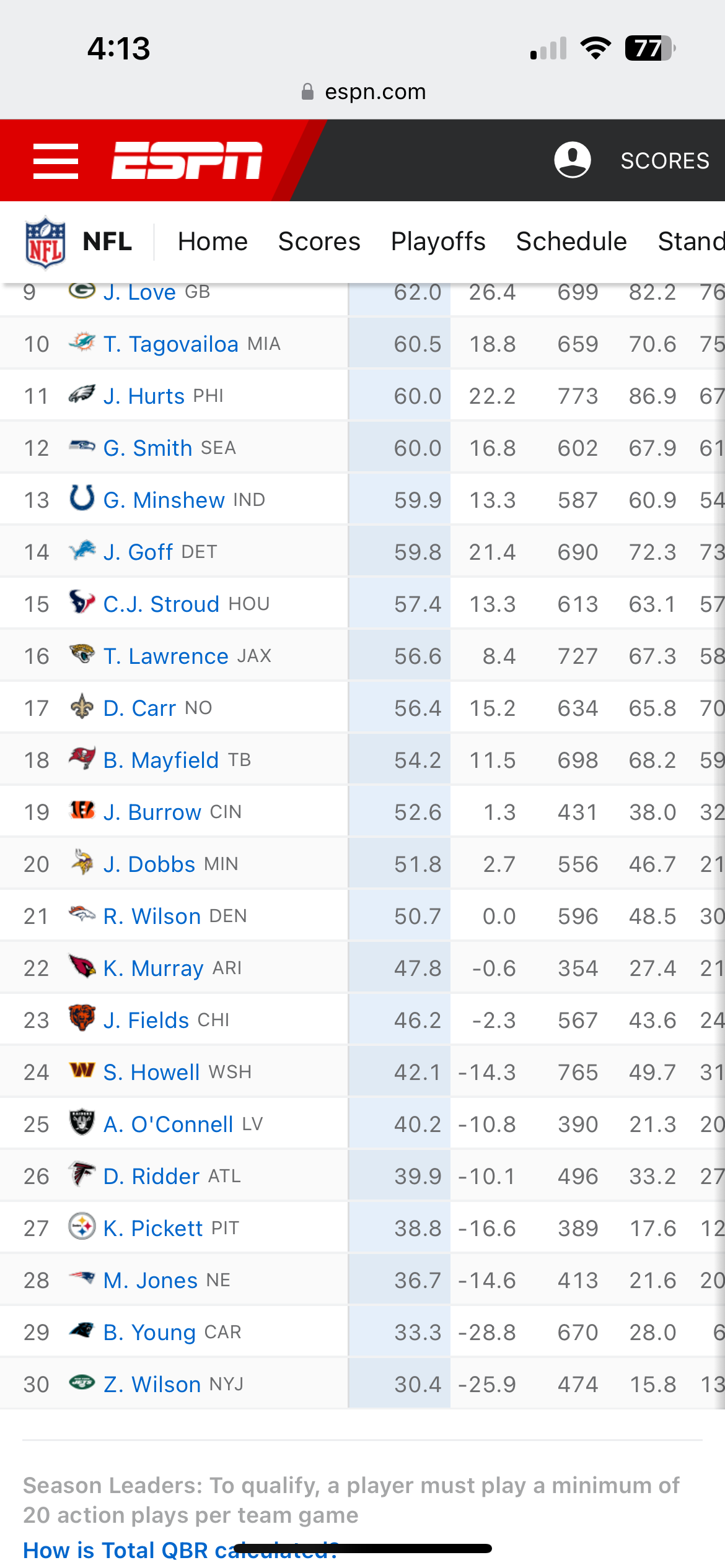The image appears to be a vertical screenshot taken from someone’s smartphone, either an Android or iPhone, displaying a page from ESPN.com. At the very top of the image, a large gray status bar is visible. On the upper left of this bar, "4:13" is displayed, indicating the time. In the middle section, there is a security padlock icon in gray. To the right of this icon, in black letters, "ESPN.com" is written. Adjacent to the URL, there is a poor Wi-Fi signal indicator, and a battery symbol showing "77%" battery life remaining.

Below the status bar, there is a long horizontal navigation bar. The left third of this bar is red and features three white bars. To the right of these bars, the ESPN logo is visible against a maroon diagonal background. The remaining part of the bar is black with an avatar icon featuring a white circular border. Inside the circle, there is a black chest symbol with a white top.

Immediately below this navigational bar is a white strip bearing the NFL logo followed by the letters "NFL" in black. To the right of this, there is a faint vertical gray bar. There are multiple options available in black letters: "Home," "Scores," "Playoffs," "Schedule," and partially cut off, "Stand."

The main content of the screenshot shows a ranked list of NFL players, starting from rank 9 and ending at 30, suggesting the user was scrolling down through the rankings. Each entry provides the player's rank, their team logo, first initial, and last name, followed by the team abbreviation in gray letters. Each row displays statistical data in decimal format. The top row of stats is highlighted in a faint blue, while the visible rows beneath each show different sets of numbers in a similar format. For instance, for rank 20, there is a Minnesota Vikings logo, "J. Dobbs" in blue letters, "MIN" in gray letters, followed by their corresponding stats.

At the very bottom of the image, small gray print states: "To qualify as season leaders, a player must play a minimum of 20 action plays per team game." Blue letters below this text read: "How is total QBR calculated?" partially obscured by a black bar cutting through the word "calculated."